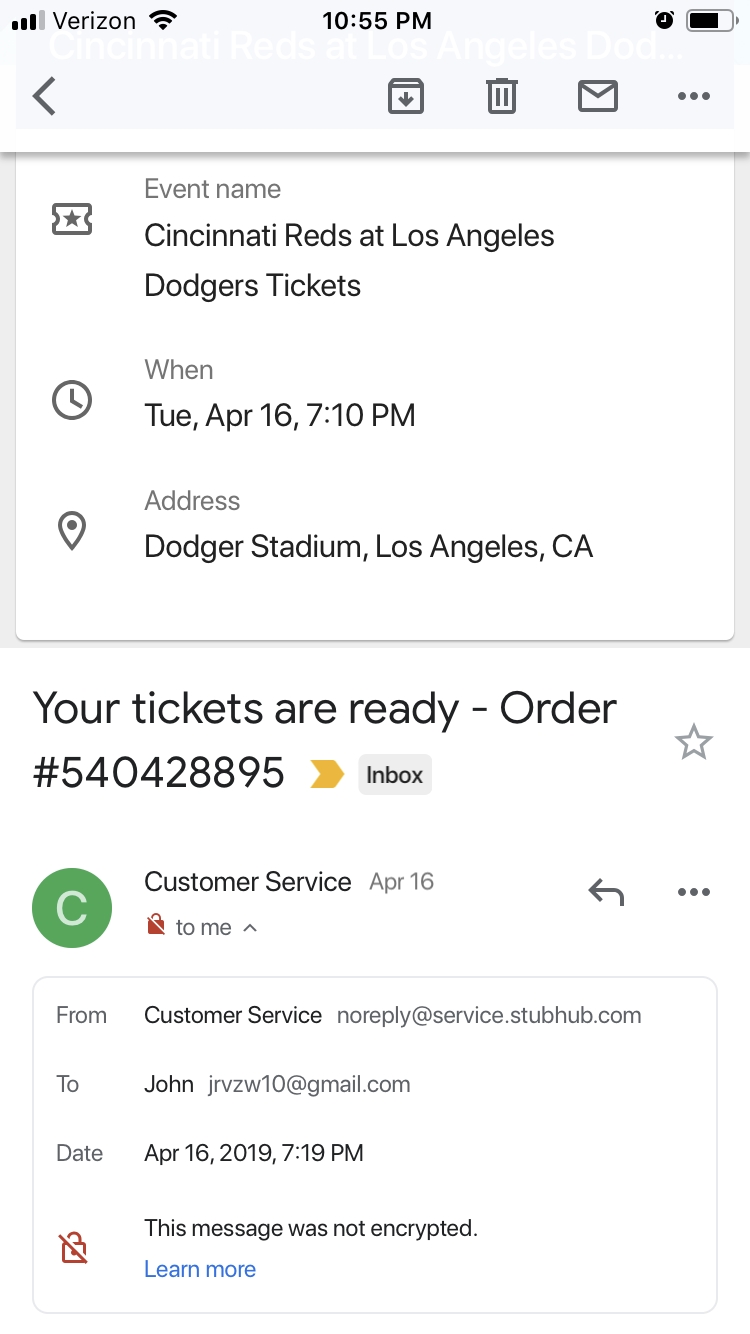Screenshot of a mobile phone display showcasing an email. 

**Top Bar:**
- On the far left: Mobile data signal icon followed by "Verizon" in black font.
- Center: Wi-Fi icon, current time displayed as 10:55 p.m.
- Right: Battery icon at half charge, alarm clock icon.

**Email Details:**
- **Subject:** Event name – Cincinnati Reds at Los Angeles Dodgers Tickets
- **Event:** Date and time – Tuesday, April 16th at 7:10 p.m.
- **Venue:** Address – Dodger Stadium, Los Angeles, CA
- **Order Information:** Your tickets are ready, Order number: 540428895
- **Indicator:** Green arrow to the right, "Inbox"

**Email Header:**
- From: Customer Service (no-reply@service.stubhub.com)
- To: johnjrzw10@gmail.com
- Date: April 16th, 2019, 7:19 p.m.
- Note: This message was not encrypted (with a learn more link).